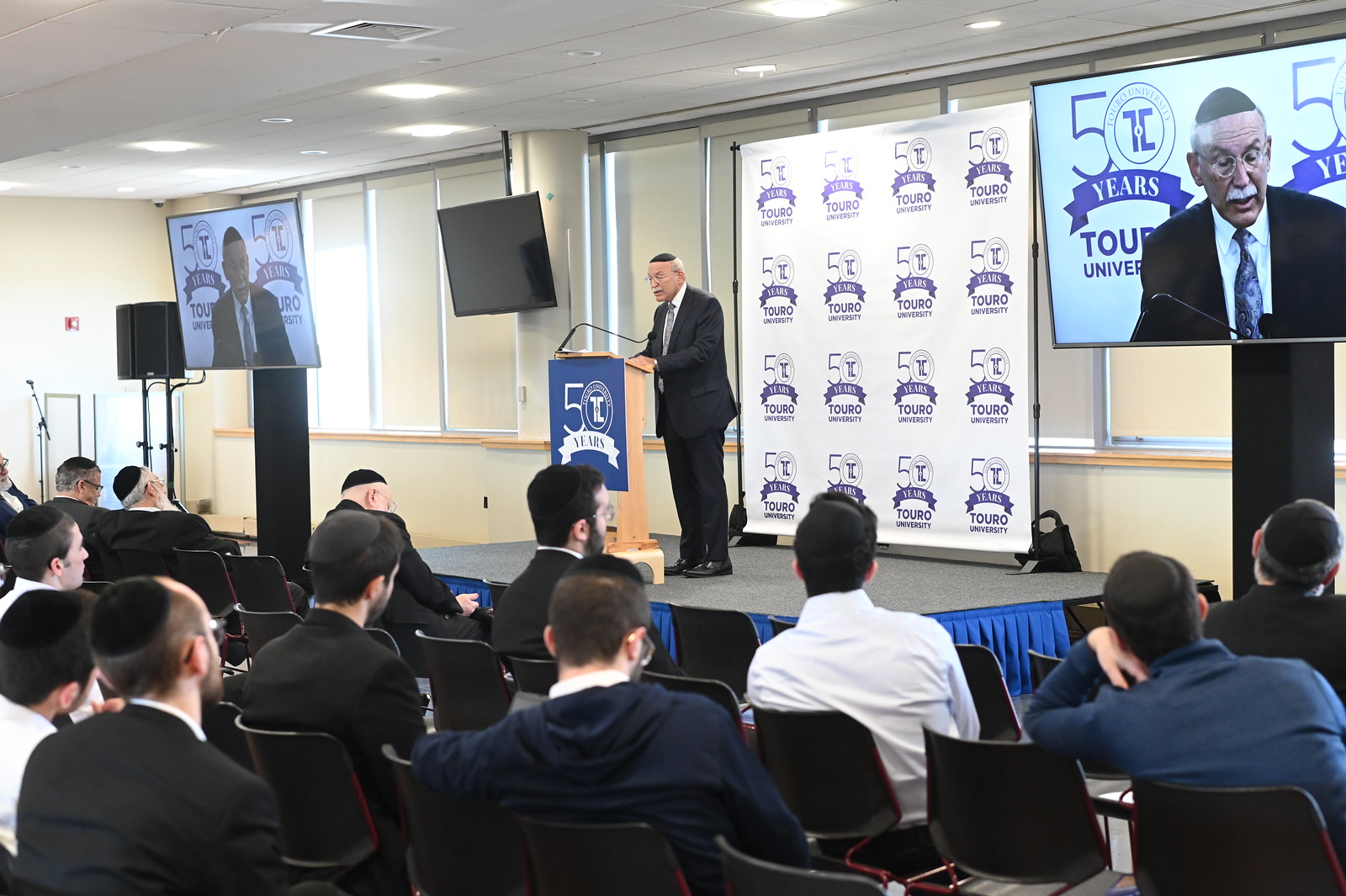An older gentleman with gray hair, a mustache, wireframe glasses, and a yarmulke stands at a wooden, elevated podium adorned with a blue banner that reads "50 years Touro University." He wears a black suit with a gray tie and addresses a gathering of young men seated in several rows of black chairs. The audience members, also wearing yarmulkes and dressed in dark sport or suit coats with white shirts, exhibit a mix of attentiveness and distraction. Behind him, large screens display his image, and the back wall features banners proclaiming "50 years Touro University," alongside windows with their shades drawn. The setting is indoors with the podium centrally located, and the event appears to be a formal lecture or presentation at Touro University.